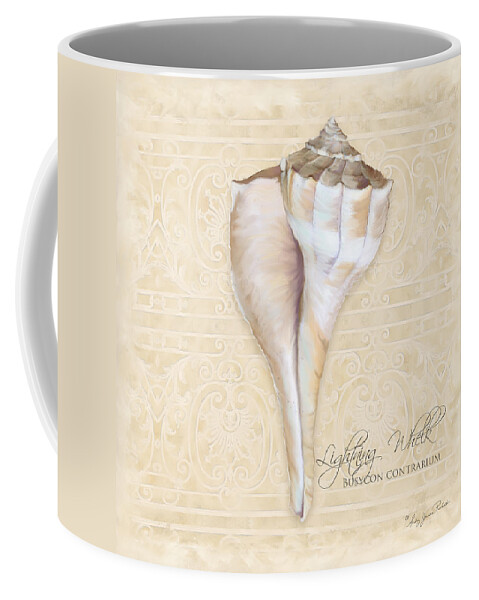The image shows a close-up of a sturdy ceramic coffee mug with a sleek, cylindrical design. The mug has straight sides and is predominantly a creamy tan color with hints of a pale peachy pink, featuring subtle, faint rococo-like designs in the background. The interior of the mug is light gray. The handle, positioned towards the left rear of the photo, is partially visible and is white in color. 

The focal point of the mug is an elongated, slender seashell design, specifically a lightning whelk, standing vertically from the base to the rim. The seashell, depicted in shades of white and tan with brown highlights towards the top, showcases intricate curved details reminiscent of its naturally occurring form. Just to the bottom right of the seashell, there is an artist's signature in thin-script black lettering, with some additional, somewhat indistinct text beneath it. This intricate mug is likely appealing to beach lovers and admirers of coastal themes.